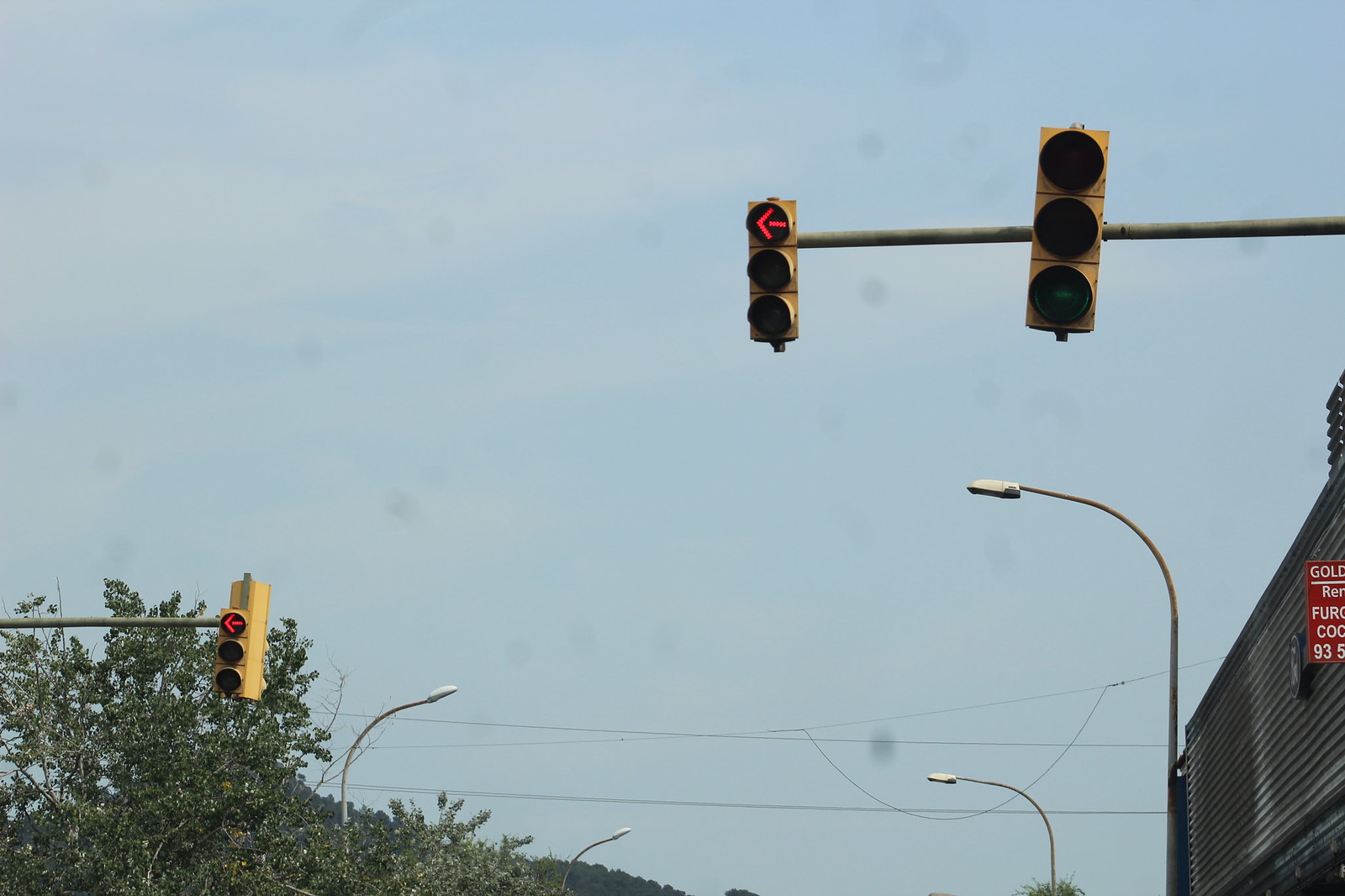In this photograph, we are looking up from ground level at a cluster of traffic signals against a cloudy, slightly rainy sky with hints of blue. Central to the image is a traffic signal with a red left-turn arrow at the top, while its middle and bottom lights are unlit. This signal is on a pole connected to another inactive light. Off to the left in the distance, another traffic light also displays a red arrow, indicating no left turn. Both of these signals face the same direction, suggesting they control the same turn at an intersection. Power lines stretch across the scene, and various street lights peak out amid the treetops. At the right edge of the image, part of a two or three-story brick building is visible, featuring a partially cropped sign with the word "gold." Water droplets on the camera lens hint at the rainy conditions, contributing to the overall grayish tone of the day.